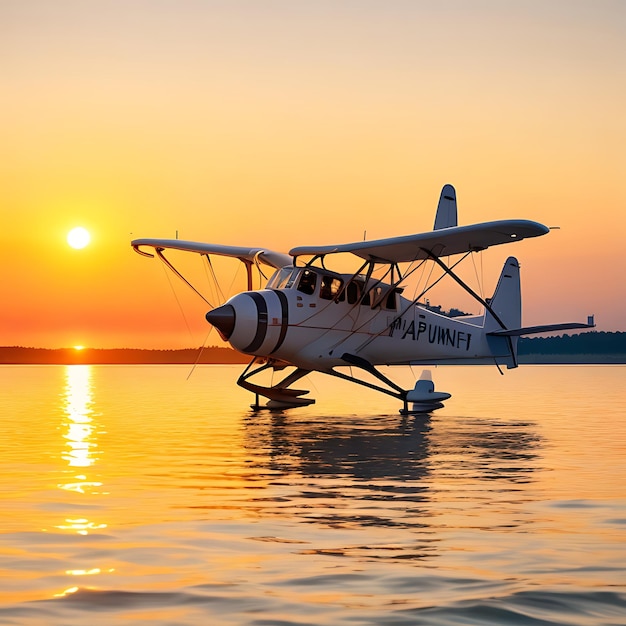This photograph presents a striking image of a white seaplane, accentuated by black detailing on its nose and black stripes around its body, floating on a calm, reflective body of water. The registration number "A-P-U-W-N-F-I" is visible on the side of the plane. The plane is angled to the left, with its nose turned slightly toward the viewer. It rests on the water, creating faint ripples beneath it. 

The backdrop features a stunning sunset, casting an orange and red hue across the entire sky, with the sun appearing as a bright, glowing yellow orb. The sun's reflection shimmers on the water, enhancing the overall scene. In the distance, there is a landscape of trees and hills silhouetted against the vivid sky; the trees on the right side appear darker, creating a contrast with the brightly lit left side. The serene setting and intricate details capture a moment that hints at either the dawn of a new day or the peaceful conclusion of one.